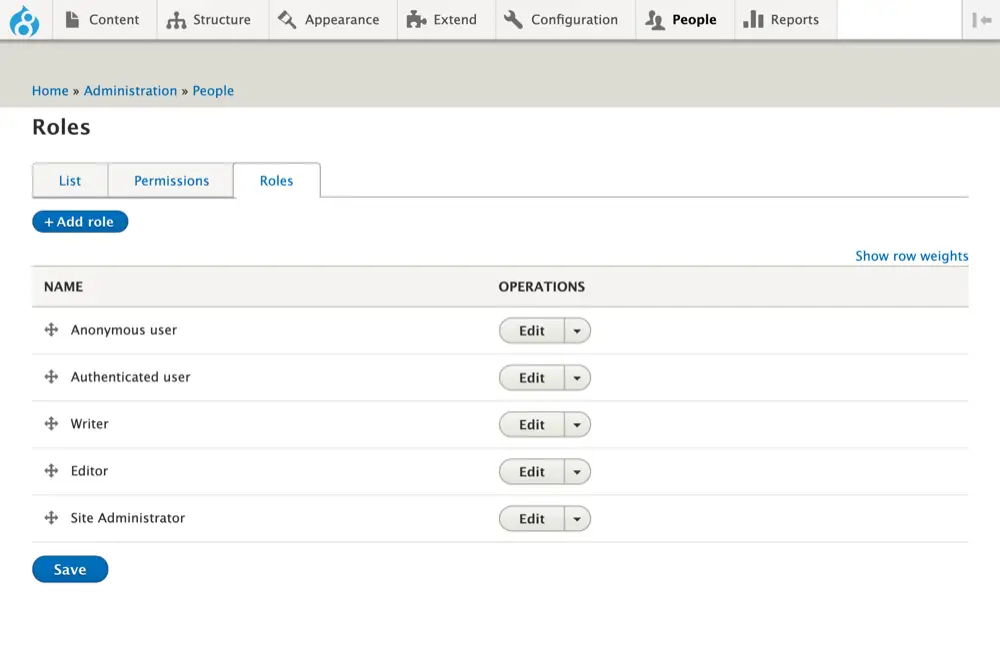The image appears to be a screenshot of a user interface from a content management or administrative web application. At the top of the interface, on a light gray background, a black font displays several tabs: "Content," "Structure," "Appearance," "Extend," "Configuration," "People," and "Reports." 

On the far left of these tabs, there's an icon resembling a water droplet with a gray figure-eight in negative space against a blue background. Below this, a darker gray strip spans the screen, with "Home," "Administration," and "People" written in blue on the left side.

Underneath, set against a white background, the word "Roles" is displayed in black. This section contains additional tabs: "List," "Permissions," and "Roles," with "Roles" being the highlighted, active tab. 

In the same area, a blue button labeled "Add role" with a plus sign in white font is present on the left side. Below this button is another gray strip with "Name" on the left and "Operations" on the right.

Following this, there is a list of roles shown against a white backdrop, each accompanied by an "Edit" button with a drop-down menu. The roles listed are "Anonymous user," "Authenticated user," "Writer," "Editor," and "Site administrator," each followed by their respective "Edit" buttons, though none of the buttons have any options currently selected from the drop-down menu.